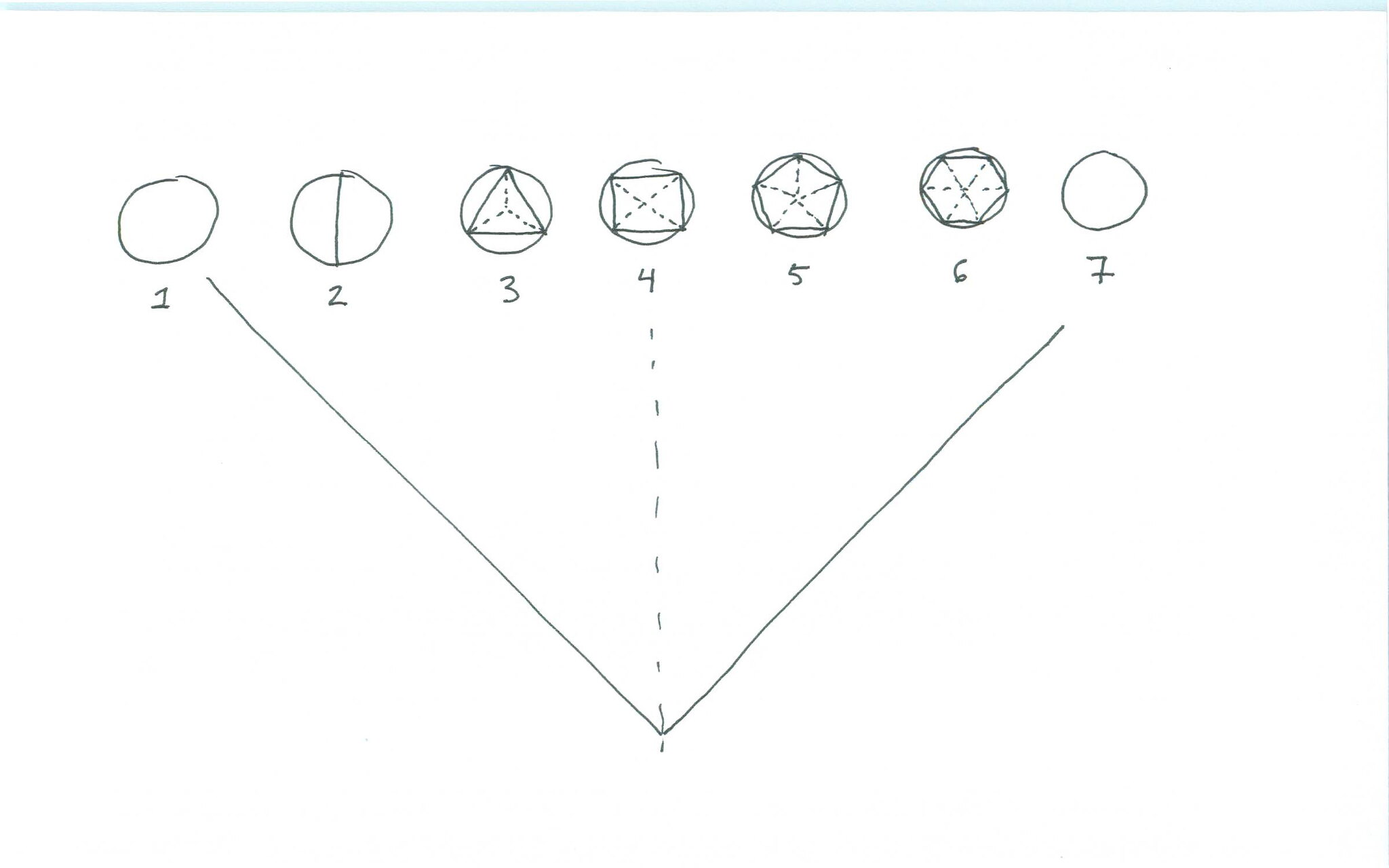The image features a white sheet of paper showcasing seven different geometric drawings, all incorporating circles. Each geometric figure is clearly labeled and distinct in its design:

1. The first drawing, labeled "1", is a simple, unembellished circle.
2. The second drawing, labeled "2", displays a circle divided vertically into two equal halves.
3. The third drawing, labeled "3", presents a circle containing a three-dimensional rectangle within it.
4. The fourth drawing, labeled "4", features a circle with a square box situated inside.
5. The fifth drawing, labeled "5", includes a circle encompassing a five-sided pentagon.
6. The sixth drawing, labeled "6", depicts a circle housing a seven-sided polygon, known as a heptagon.
7. The seventh drawing, labeled "7", mirrors the first circle as another plain, empty circle.

Each circle is meticulously drawn and showcases a progression from simple to more complex geometric shapes.